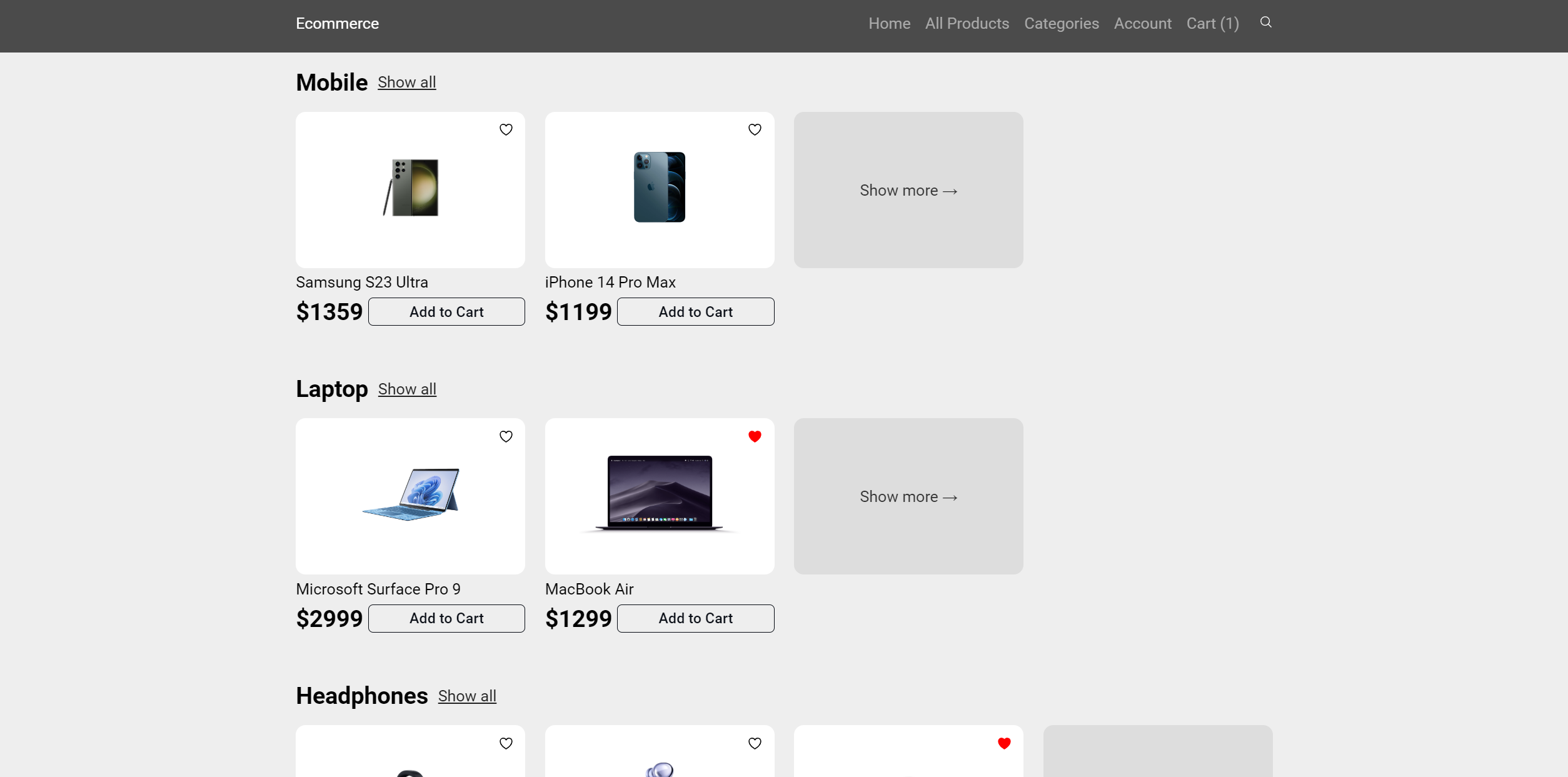The image displays a screenshot of an e-commerce website featuring an off-white background. At the top, there's a dark gray horizontal bar with "e-commerce" written in small white text on the left. On the right side of the bar, navigation options such as Home, All Products, Categories, Accounts, and Carts are listed. 

The main section of the webpage showcases four images of various mobile devices. In the upper left corner, there is a smartphone priced at $1,359. Adjacent to it on the upper right is another smartphone priced at $1,199. On the lower left, a laptop is featured with a price tag of $2,999.